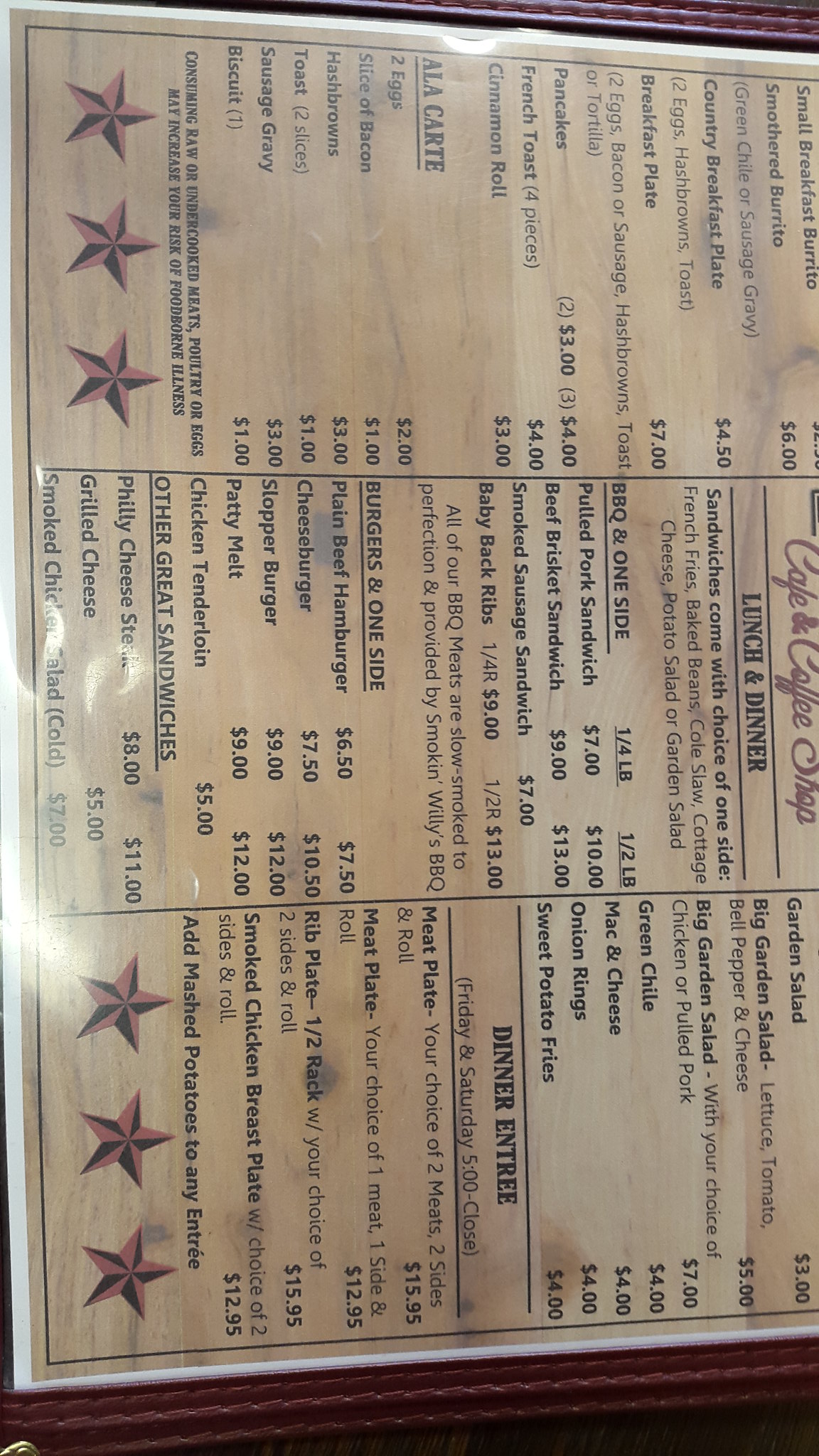This image captures a detailed photo of a glossy, wooden-themed menu from a cafe and coffee shop. The menu appears to be positioned sideways, requiring the viewer to tilt their head to read it properly. The menu is divided into three columns:

**Left Column (Breakfast Items):**
- **Small Breakfast Burrito:** $6
- **Smothered Burrito:** $4.50
- **Country Breakfast Plate:** Available with either green chile or sausage gravy, $7

The background features a high-gloss finish, suggesting it is either laminated or printed on glossy paper. At the bottom of the left column, decorative red and black stars, each split into a two-tone pattern, accentuate the menu's border.

**Middle Column (Lunch and Dinner):**
- This section is headlined by "Lunch and Dinner" in prominent black text, mentioning that sandwiches are served with a choice of one side.
- **Available Sides:**
  - French Fries
  - Baked Beans
  - Coleslaw
  - Cottage Cheese
  - Potato Salad
  - Garden Salad
- **BBQ Pooled Pork Sandwich:** Priced at $7 and $10, with two columns indicating different portion sizes or options.

The middle column also features glossy background and star decorations similar to the left column.

**Right Column (Additional Food Options and Dinner Entrées):**
- **Garden Salad:** $3
- **Big Garden Salad:** Includes lettuce, tomato, bell pepper, and cheese, $5
- **Dinner Entrées:**
  - Separated by two lines to highlight the section.
  - **Meat Plate:** Your choice of two meats, two sides, and a roll, $15.95

The entire menu is bordered in white and seems to be presented in a format similar to a table menu, possibly slipped into a menu binder. The overall layout is long and rectangular, making it easy to hold and read at a table.